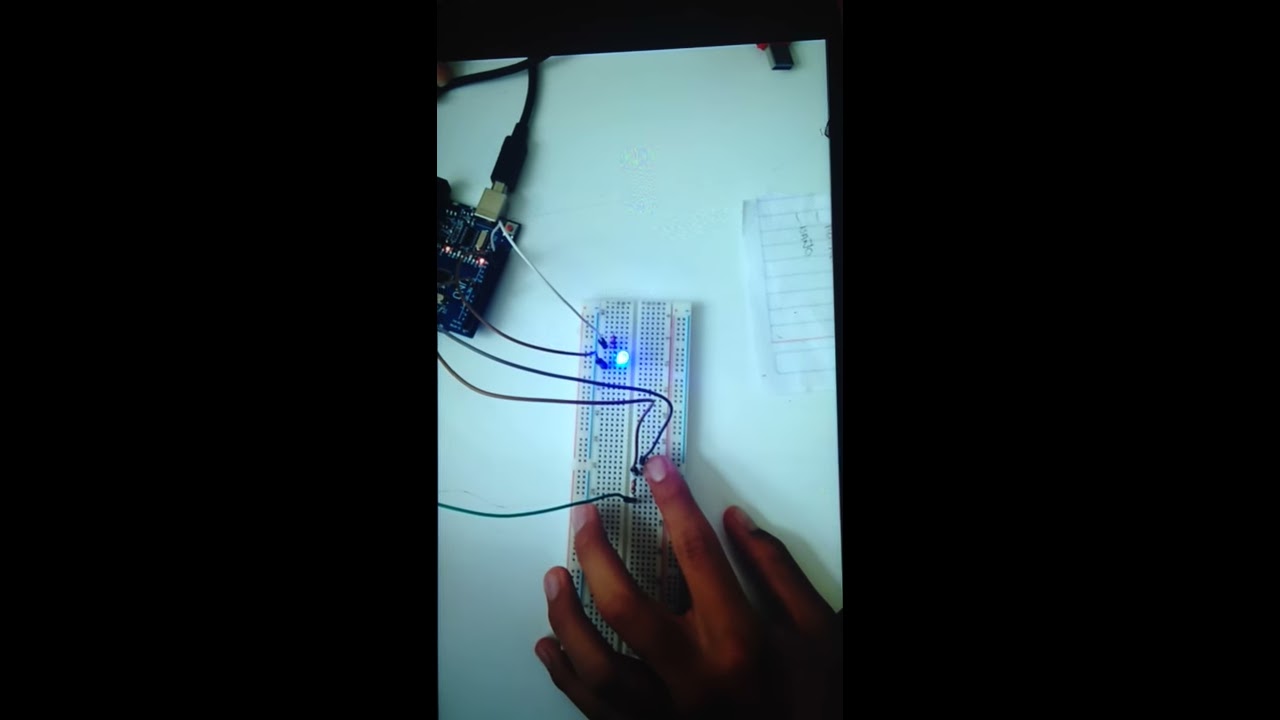The image shows a detailed setup of an electronics project centered around a white rectangular electronics board. This board occupies the center of the image and features various black holes along with distinctive blue and red lines and a prominent lit blue LED light towards the top. Connected to this board are five wires leading to another electronics device on the left side of the image. This device is blue, distinguished by black chips, two red LED lights, and a silver plug connected to a black power cable. A tan-colored hand is shown in the bottom right corner of the image, pressing down on a wire on the white electronics board. Another black wire stretches across the top left corner of the image. On the right side, a piece of paper with black lines is visible, and in the very top right corner, there is a USB plug. The scene is set on a white desk, framed by large black rectangle borders on the left and right.